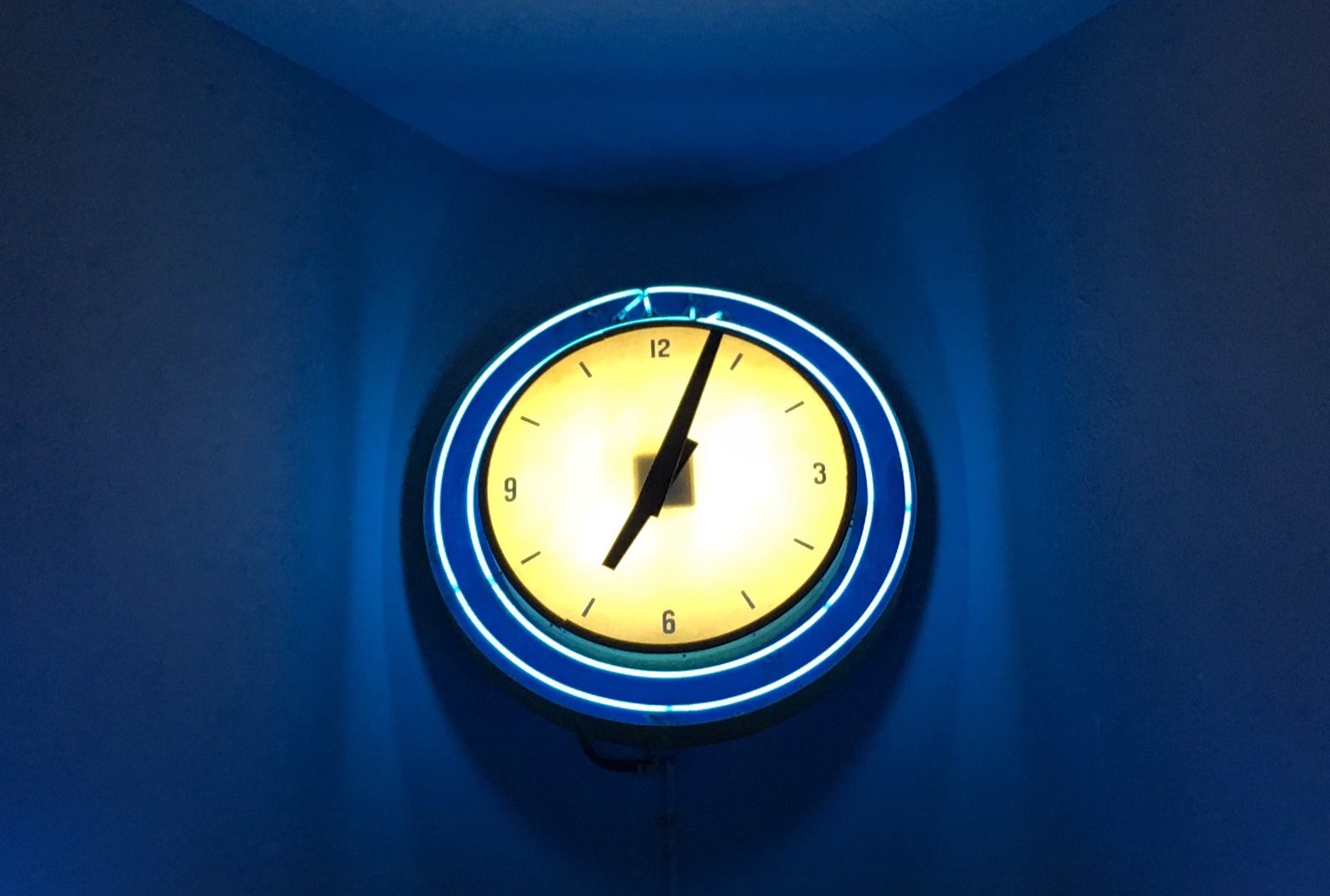In this image, we see a blue wall accented with varying shades of blue, influenced by the lighting emanating from a central wall clock. The clock, prominently lit in the middle, features a thin strip of neon light encircling its diameter and another strip outlining its face, both in a striking white hue. The clock itself is also blue, creating a harmonious blend with the wall. The face of the clock is a yellowish color, with the hours twelve, three, six, and nine clearly marked. Simpler black lines denote the other hours. The lighting from the clock casts an intriguing play of light and shadow across the wall, with darker shadows appearing on both the right and left sides. Primarily, the light radiating from the clock illuminates the narrow strips directly to its right and left, as well as the areas above and below it, adding to the captivating visual effect.